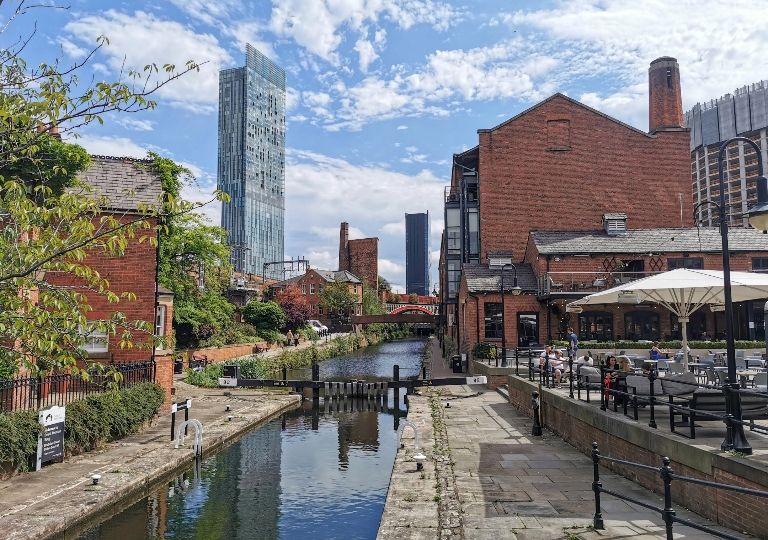The image is a large, almost square-shaped horizontal photograph showcasing a picturesque city scene. At the top, the sky is a clear blue, adorned with feather-like white clouds. Central to the image is a narrow, calm canal of bluish-gray water, bordered by stone walls on either side. 

On the right side, there's a notable outdoor dining area enclosed by metal bars, equipped with gray cushioned seats and prominently featuring a large white umbrella. People are seated at the tables, giving the place a lively atmosphere. Adjacent to this seating area is a tall, three-story red brick building, possibly a restaurant, with balconies and a big chimney extending from its backside. Further behind this structure, another larger building rises, hinting at an even grander urban landscape.

To the left of the canal, a smaller red brick building with a gray roof stands, partly obscured by a large tree. Scattered trees and patches of grass add a touch of greenery to this side. The background reveals a series of old brick buildings, complementing the historical charm of the scene, while two massive skyscrapers loom further out, their reflective surfaces strikingly juxtaposed against the older architectures.

Completing the scenic view, a couple of small bridges span the canal in the far distance, adding to the overall quaint, yet vibrant, impression of the city.